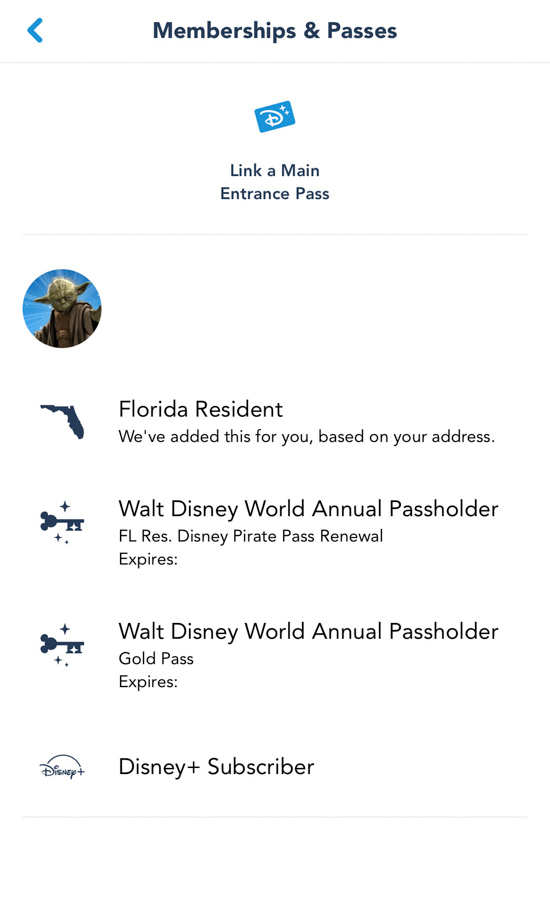This is a detailed screenshot from a website or application designed in a mobile-friendly format, identifiable by its narrow layout and absence of standard browser or device UI elements. The interface rests on a clean, white background.

At the top of the screen, bold dark blue sans-serif text reads "Membership and Passes." To the left, a light blue arrow icon is positioned, signifying a navigational element. Below this title, a thin, light gray line approximately two pixels wide separates the header from the subsequent sections.

The following section features a small rectangular element resembling a gift card, adorned with a light blue background and a white Disney logo. Below this graphic appears the text "Link a main entrance pass." Another light gray divider line follows, maintaining consistency in the design.

The next substantial section displays a circular image of Yoda, likely functioning as a user avatar or related graphic. Underneath, there are four rows of information, each formatted with a dark blue header, subtext, and a corresponding icon.

1. **Florida Resident**: The text explains, "We’ve added this for you based on your address," accompanied by an icon of Florida on the left.
2. **Walt Disney World Annual Pass Holder - FL Res Disney Pirate Pass Renewal**: An icon of a key featuring a Mickey Mouse head and sparkles is displayed. However, the expiration date field is blank.
3. **Walt Disney World Annual Pass Holder - Gold Pass**: Again, an icon of the Mickey Mouse key is present, but the expiration date section is empty.
4. **Disney Plus Subscriber**: This row includes a simple Disney icon.

The interface concludes with one final thin light gray divider line at the bottom, neatly segmenting the end of the content.

Overall, the design leverages a clean, minimalistic aesthetic, with consistent color usage and clear sectioning to enhance readability and user experience.